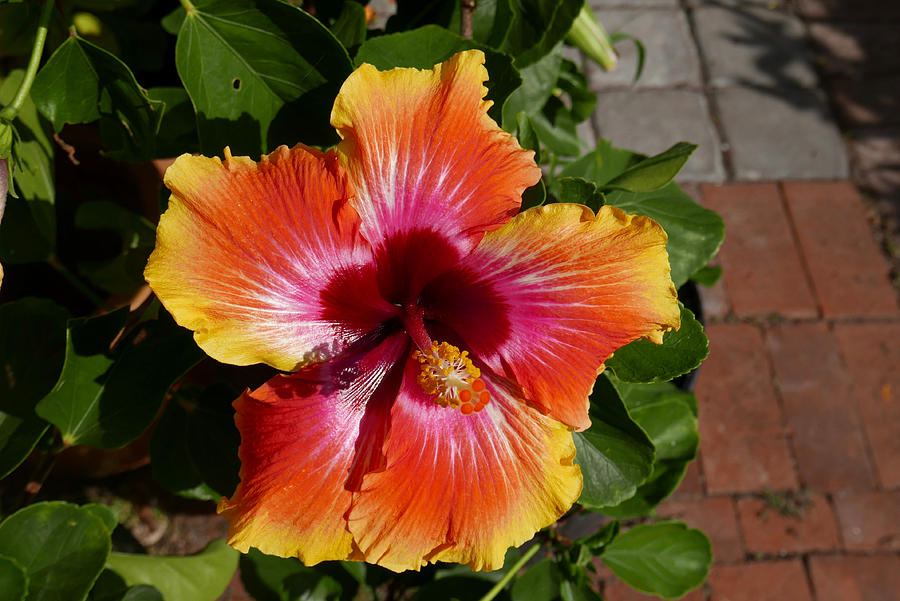In the image, taken on a sunny day, a vibrant lily blooms at the center, serving as the focal point amidst lush green leaves. The lily's five petals exhibit a stunning gradient—starting with bright yellow tips that transition into a rich orange and finally blending into a vivid pink towards the innermost part. The flower’s heart showcases a central stalk adorned with yellow pollen, adding to its intricate beauty. The dark green leaves surrounding the lily have natural imperfections, including a small hole in one at the top. To the right, a garden walkway is visible; the lower portion is lined with red brick pavers, while the upper portion features smaller, gray square pavers, framing the floral spectacle perfectly.